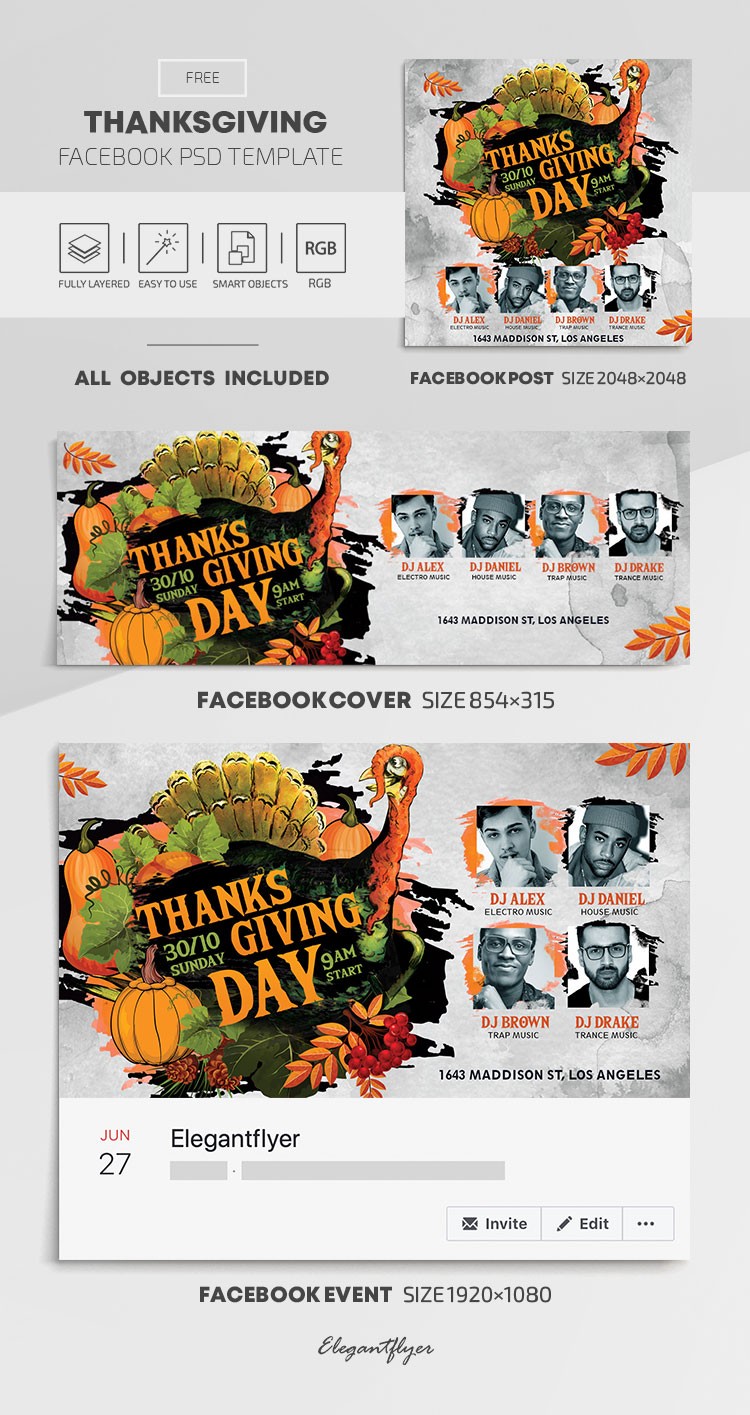Caption: 

On a sleek grey background, this comprehensive flyer template for a Free Thanksgiving Facebook PSD template offers a vibrant and organized layout. 

In the upper left-hand corner, bold text announces the "Free Thanksgiving Facebook PSD Template." Prominently featured is a festive turkey illustration in autumn colors of brown, green, yellow, and orange. Below this illustration are images of four men of different races, each positioned distinctly.

Further down, the template showcases a suggested Facebook cover design with dimensions clearly stated as 854 x 315. This cover prominently displays the same colorful turkey along with a notable message in large red font: "30/10 Sunday, Thanksgiving Day." The images of the four men—DJ Alex, DJ Danielle, DJ Brown, and DJ Drake—appear again in a slightly varied arrangement.

At the bottom of the flyer, within a crisp white rectangle, the text "Elegant Flyer, June 27th" is displayed, followed by additional specifications for a Facebook event design with a size of 1920 x 1080 pixels. The template is signed off with the brand mark "Elegant Flyers," lending an air of professionalism and quality to the overall design.